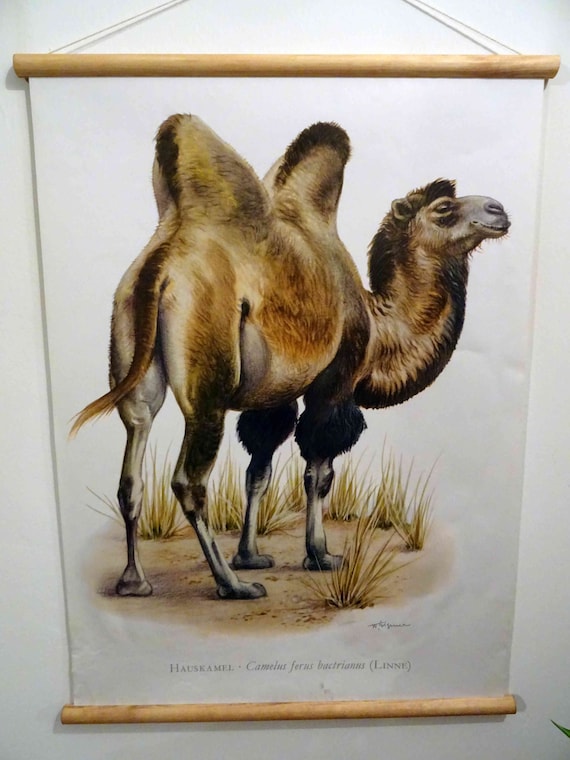The image depicts a portrait-oriented, color photograph of a banner illustrating a camel. The banner hangs on a light gray wall, suspended by a white string attached to two round, light brown wooden dowels at the top and bottom edges, creating a scroll-like appearance. The camel, centrally positioned and viewed in profile facing the right side, features two prominent humps extending in opposite directions from its back. It has a curving neck covered in dark brown fur, leading to a head with closed eyes and a mouth that is gray in color. The top segment of the camel's legs is black, transitioning to lighter hues with a segmented appearance. The camel stands on a dirt patch interspersed with tall, beige grass clusters. The background of the banner itself is white, complementing the detailed illustration. At the bottom, the banner includes the text "House Camel" followed by "Camellius Ferris Bactrians."